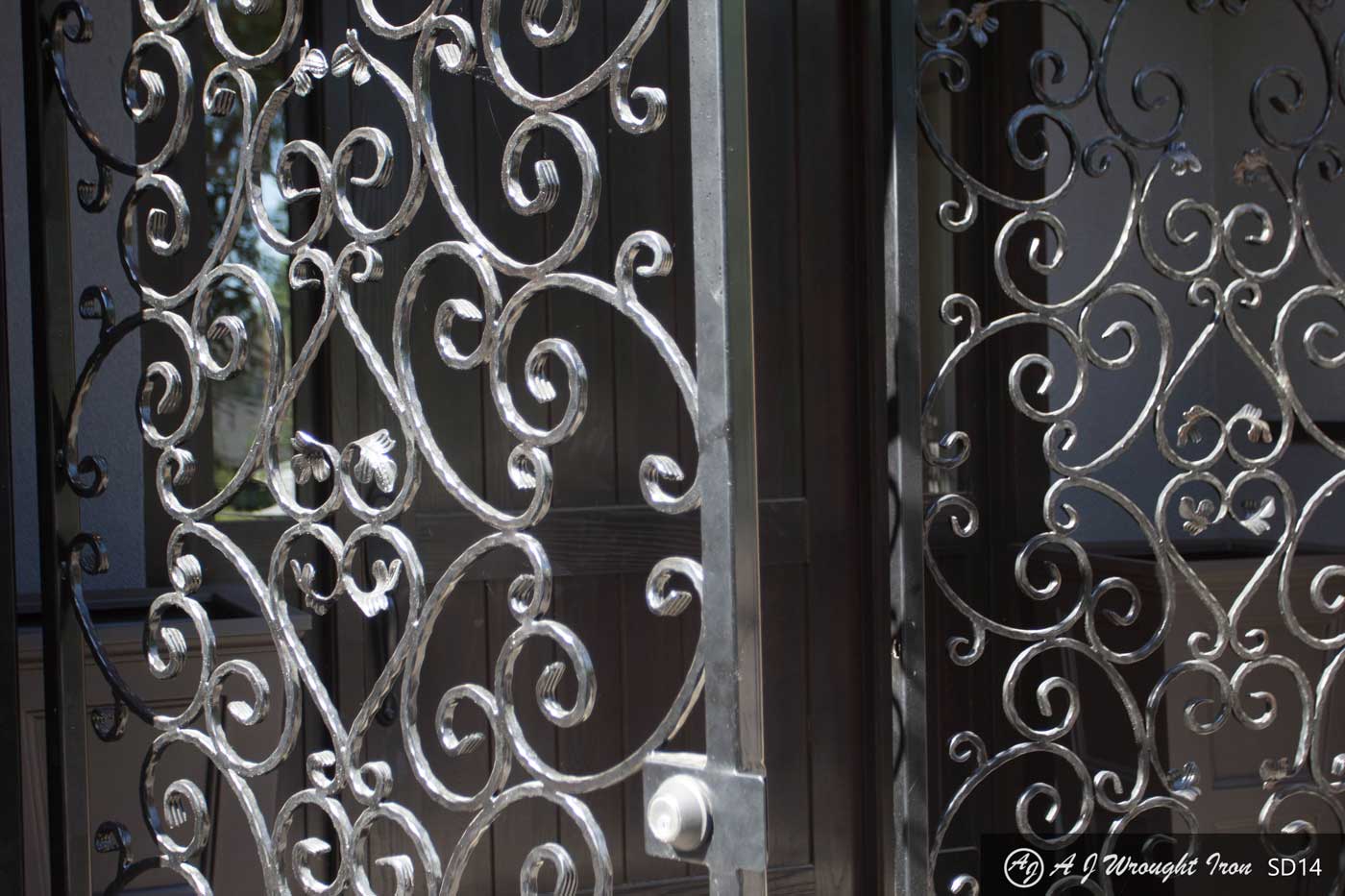This image captures a pair of slightly open wrought iron gates, chrome in color, mounted outside a house or building. Each gate half is intricately designed with ornate curling patterns and appears robust and secure, crafted from shiny steel or unfinished iron. The gate on the left features a round handle mounted on a brass or silver plate, while the one on the right, although mostly closed, has a shadow cast on it due to the slight opening of the left gate. Blue walls and a large wooden door can be seen through the gates. The bottom right corner of the image displays a white emblem with the letters "A" and "G" at the center, accompanied by the inscription "AJ Roth Iron SD14."